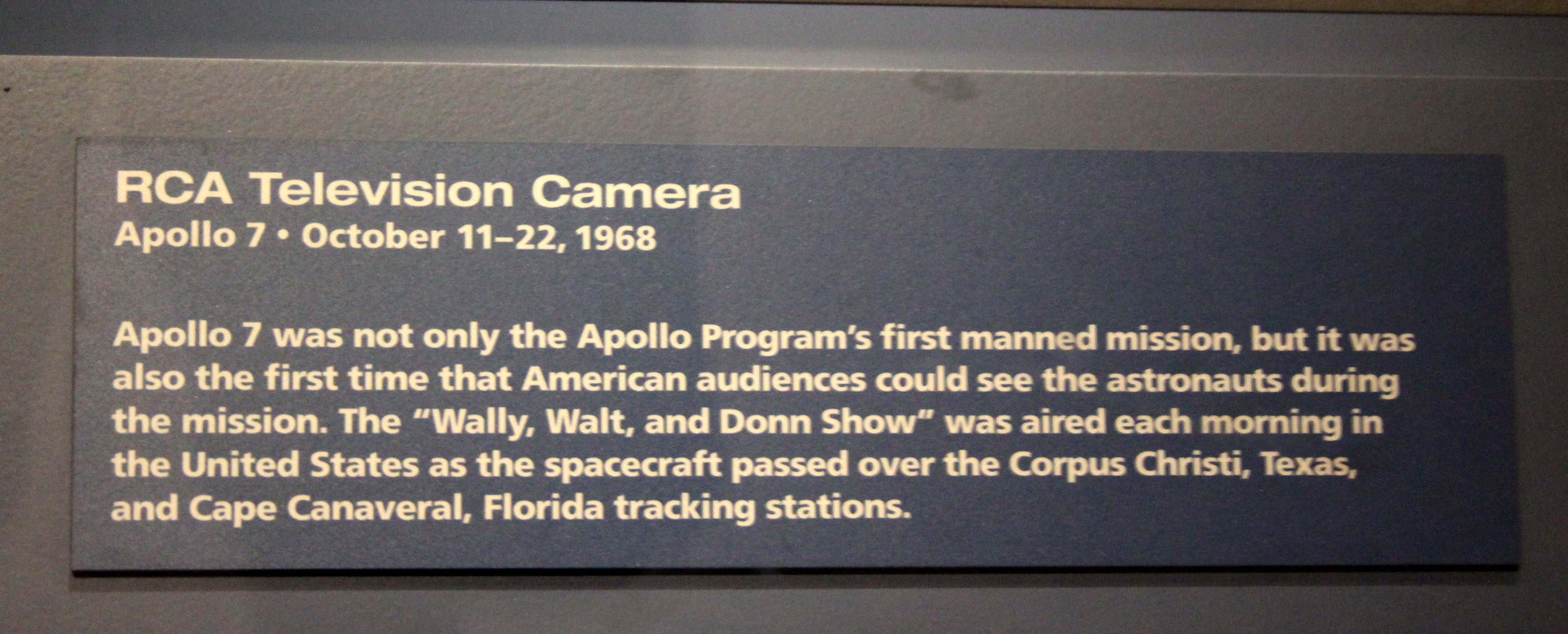The image showcases a close-up view of a blue descriptive plaque, likely set in a museum, against a gray, possibly plastic backdrop. The plaque, centered in the image, bears white text that reads: "RCA Television Camera, Apollo 7, October 11-22, 1968." The plaque provides historical context, noting that Apollo 7 was the Apollo program's first manned mission and the first occasion where American audiences could see astronauts live during the mission. It highlights the significance of the "Wally, Walt, and Don Show," which was aired each morning as the spacecraft passed over the tracking stations in Corpus Christi, Texas, and Cape Canaveral, Florida. The colors in the image are predominantly black, gray, and tan, emphasizing the plaque's importance and its informative role in the display.